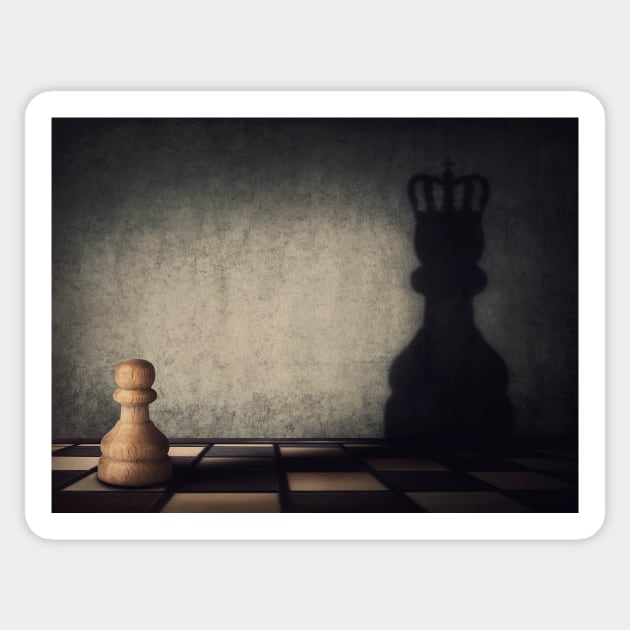The image depicts a dimly lit painting bordered by a thick white frame, presenting a detailed and atmospheric scene. The foreground features a chessboard with black and tan squares, of which about five squares run horizontally and vertically. In the lower left corner of the chessboard sits a charming pawn chess piece made of light tan wood, resting on a white square. The background reveals a dark, possibly gray wall that contrasts with a distinct, large shadow of what appears to be a king or queen chess piece. This shadow, noticeable due to a faint spotlight, stretches from the bottom right up the wall, enhancing the enigmatic ambiance of the scene. Light emanates softly from the left, casting subtle shadows and making the right side appear darker. The entire composition is encapsulated by a gray background, emphasizing the mysterious and reflective nature of the artwork.